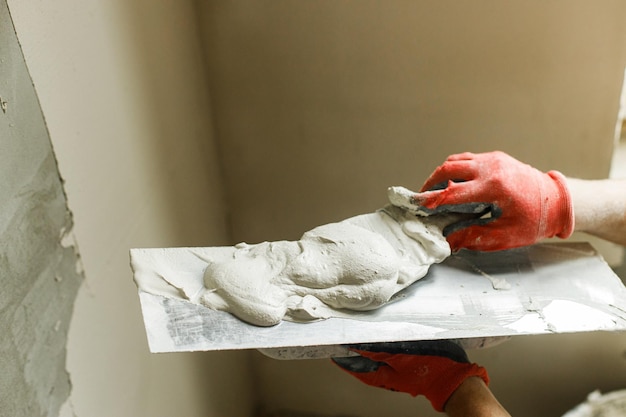In this detailed image, a plasterer is diligently working on a corner section of a wall. The plasterer, identifiable only by their forearms and hands, is seen wearing red gloves with black inner hand sections. The gloves are vivid and well-defined against the grey wall they are working on. The person is using a trowel, a flat rectangular tool, to apply light grey plaster onto the wall, which has already undergone some initial plastering. Their hands are meticulously handling the freshly mixed plaster, preparing to smooth it onto the surface.

The room itself appears to have beige walls, but a section to the left shows some paint peeling or intentionally removed. The focal point of the image is the hands and the actions of plastering, emphasizing the careful and precise movements required in the trade. The surrounding area fades into the background, highlighting the concentrated effort of the plasterer as they bring the wall closer to completion. The scene captures a moment of skilled craftsmanship, with the plasterer methodically working to perfect the wall’s surface.